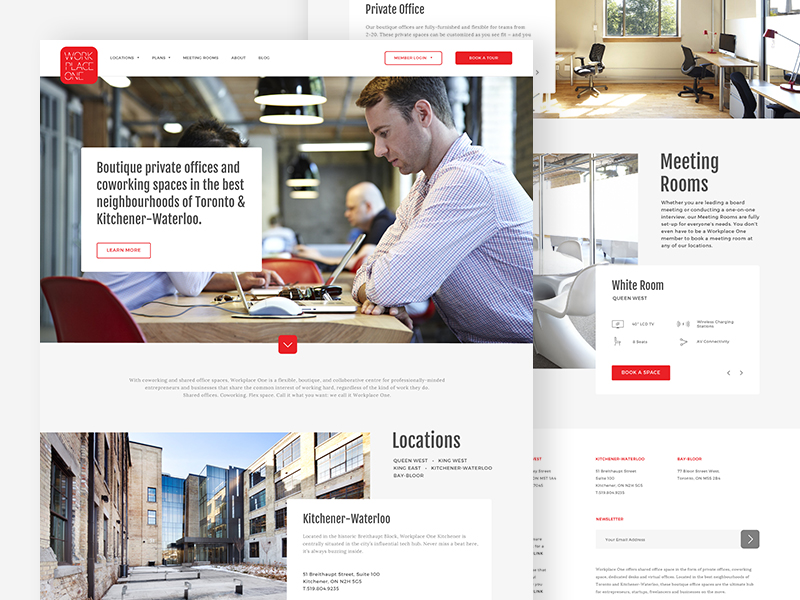The image captures two overlapping screenshots from the website "Workplace One," showcasing different sections yet belonging to the same site. 

### First Screenshot:
- **Header:** Displays the brand name "Workplace One."
- **Central Image:** Features a man sitting at a desk, engrossed in his computer, surrounded by several other individuals.
- **Text Box:** Contains promotional copy stating, "Boutique Private Offices and Coworking Spaces in the Best Neighborhoods of Toronto in Kitchener-Waterloo," with a clickable "Learn More" button below.
- **Sections:** 
  - A title labeled "Locations," featuring the first listed location, "Kitchener-Waterloo."

### Second Screenshot (Partially Obscured):
- This screenshot lies beneath the first and shows:
  - **Section Titled "Private Office:"** Accompanied by an image of a neatly arranged office.
  - **Meeting Rooms Section:** Following the office section.
  - **White Room Box:** A specific mention or feature listed below Meeting Rooms.
  - **Fine Print Text:** Additional content situated towards the bottom in smaller font, likely detailing further information or disclaimers.
  
 ### Additional Element:
- **Search Bar:** Located in the lower right-hand corner, appears to be a field for entering an email address.

This set of screenshots provides a comprehensive glimpse into the offerings and layout of the Workplace One website, emphasizing their focus on premium office and coworking spaces, with detailed visuals and navigational options.